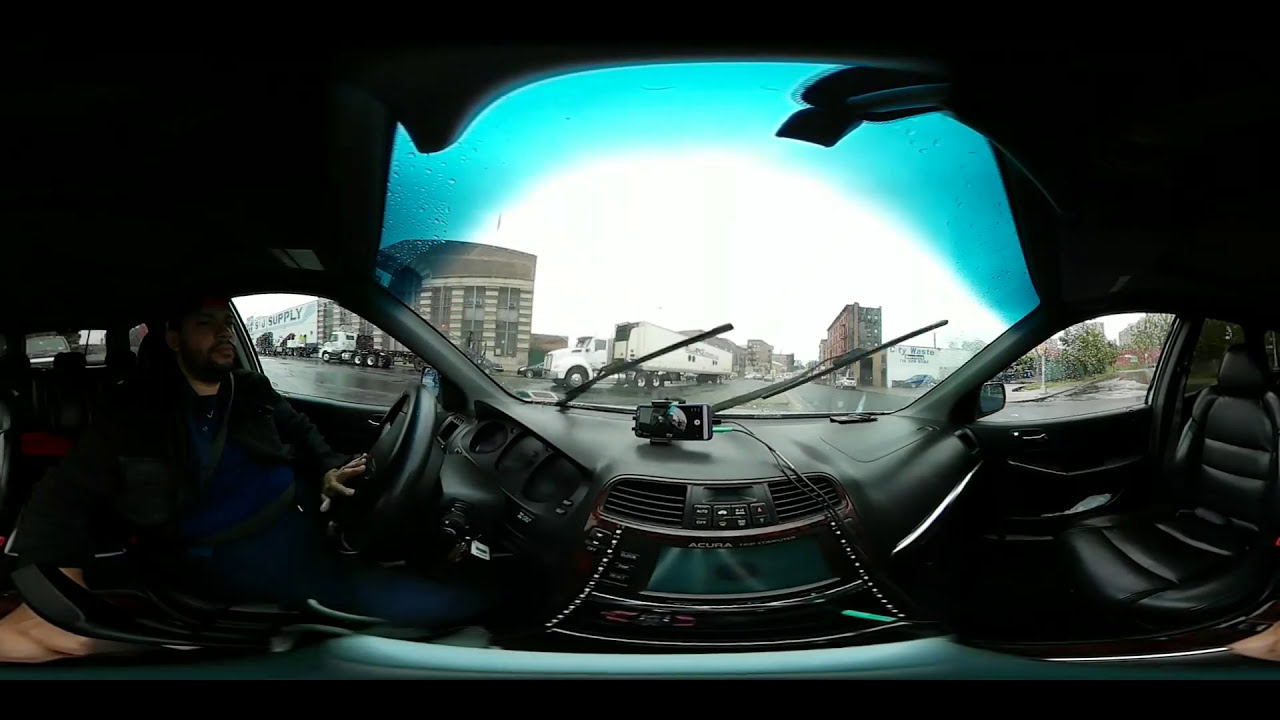The photo is a panoramic or 360-degree image taken from the interior of a car with a black interior, leading to a distorted and stretched-out effect. On the left, the driver, a Black man with a black beard, dressed in dark clothes that include a black jacket, a blue shirt, and blue jeans, holds the bottom of the steering wheel. The driver's seat faces the right side of the image. The car features a shiny black leather passenger seat on the right, which appears very clean.

In the center of the image, the dashboard is visible with the radio console prominently displayed, clearly marked with "Acura." The driver's cell phone is mounted on the dashboard for charging. A windshield wiper is in action due to the rain, adding to the blurred and white appearance of the background sky, which also shows spots of blue. Beyond the windshield, a large white tractor-trailer truck, or 18-wheeler, is seen driving on what looks like city streets. Surrounding buildings exhibit an older architectural style, suggesting a European cityscape.

On the left side of the image, visible through the driver's side window, there is a mural on the wall of a building. To the right, visible through the passenger window, another road intersects with trees and a sidewalk lining it. Through the condensation on the car windows, the panoramic view captures the city atmosphere, emphasizing the busy street scene with intersecting roads and the large truck between two buildings.